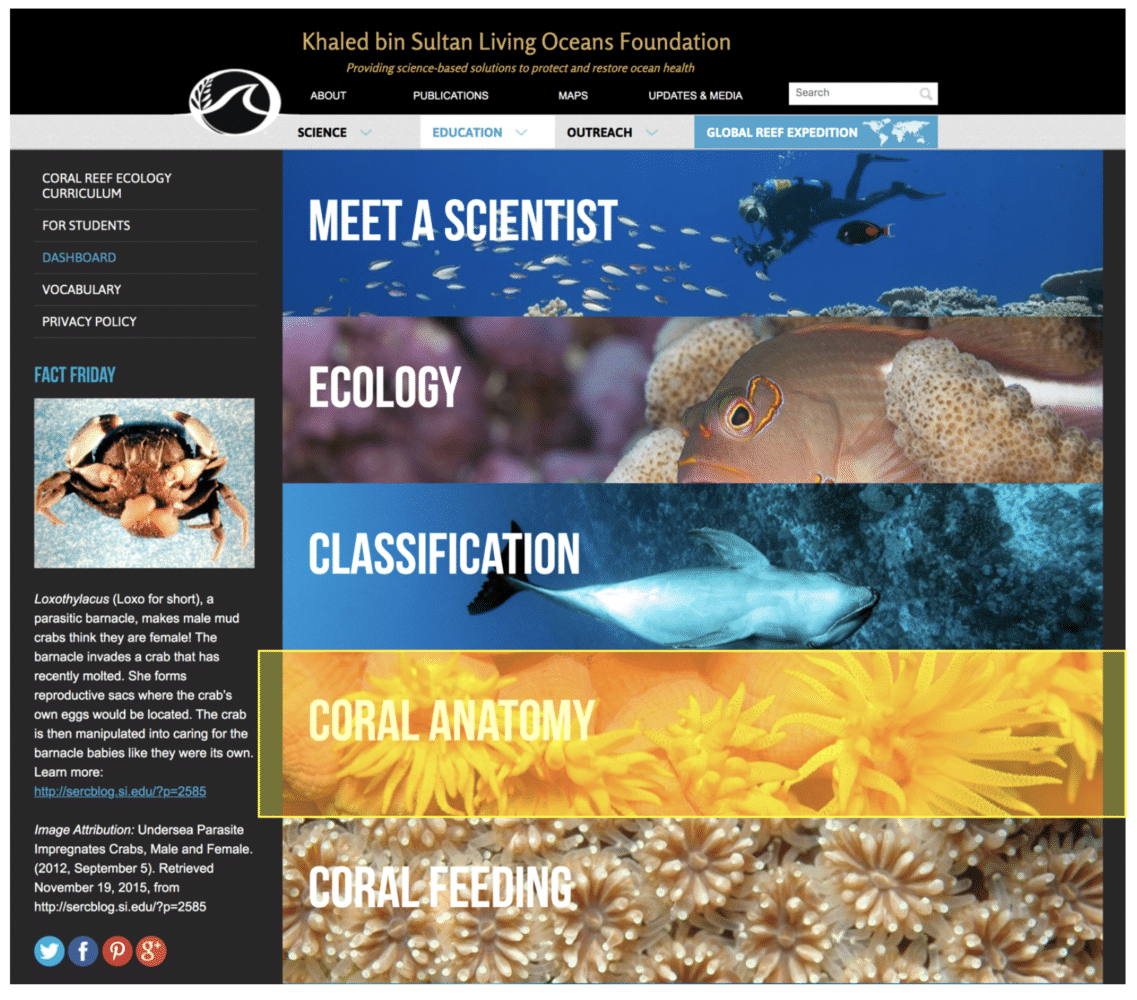"This image features the homepage of a marine-focused website dedicated to the Khalid bin Sultan Living Oceans Foundation, with a black background. At the top, the page prominently displays the foundation’s name along with its mission statement: 'Providing science-based solutions to protect and restore ocean health.' Centered near the top is a black and white logo for the website. To the right of the logo, navigation links include 'About,' 'Publications,' 'Maps,' 'Updates,' and 'Media,' next to a search bar.

Directly below, there are additional tabs labeled 'Science,' 'Education,' 'Outreach,' and 'Global Reef Expedition.' On the left sidebar, descending along the page, are tabs for 'Coral Reef Ecology Curriculum,' 'Curriculum for Students,' 'Dashboard,' 'Vocabulary,' and 'Privacy Policy.' Also listed is 'Fact Friday,' which currently features a fact about a crab.

To the right of these sections, there are categories for 'Meet a Scientist,' 'Ecology,' 'Classification,' 'Coral Anatomy,' and 'Coral Feeding,' providing various educational resources on marine life."